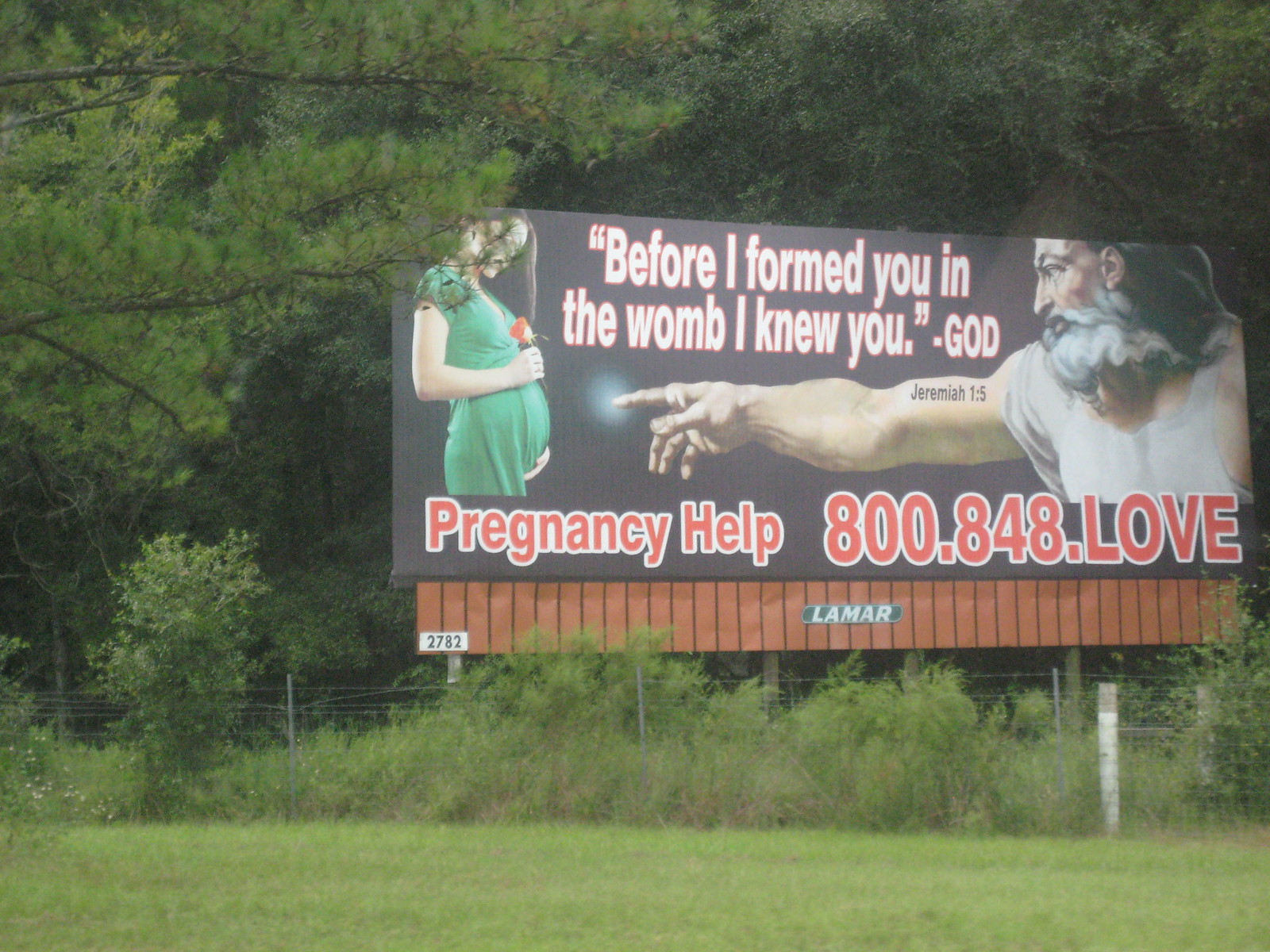This image captures a commercial billboard set against an overgrown, forest-like backdrop featuring long-limbed trees and scattered vegetation. The billboard communicates a religious message about pregnancy. At the center, it displays a quote from Jeremiah 1:5, "Before I formed you in the womb, I knew you," attributed to God. To the left, there's an image of a pregnant woman dressed in a green gown, holding a red rose and looking down. Opposite her, on the right, is a depiction of God with a billowy white beard, wearing a white robe. God's arm is outstretched, pointing towards the woman with his finger illuminated and Jeremiah 1:5 inscribed on his bicep. Below the quote, in bold red text, it reads, "Pregnancy Help: 800.848.LOVE." The billboard is framed by a wooden border and features the name Lamar Outdoor Advertising along with the number 2782. At the base of the sign, there’s a mesh wire and barbed wire fence intertwined with weeds, with a grassy field laying in the foreground.